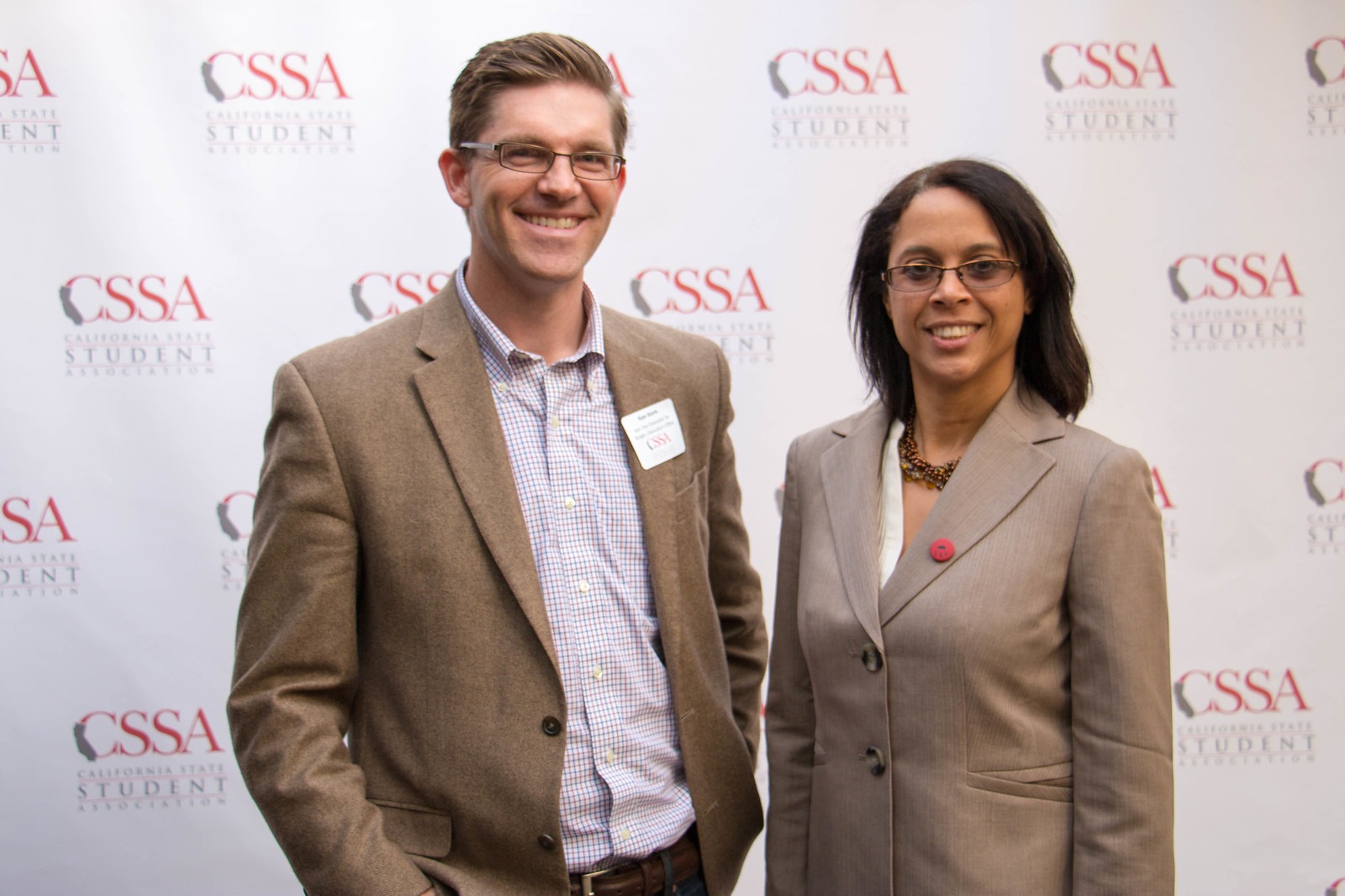In this photo, two individuals, a man and a woman, are standing side by side at what appears to be a professional event, possibly a conference or a student association gathering. The background features a repeating pattern typical of a photo backdrop, with the acronym "C-S-S-A" prominently displayed in red, alongside less legible gray text that likely reads "California State Student Association."

The woman, positioned on the right, has a radiant smile and wears glasses with a slight tint. Her attire includes a tan or khaki professional jacket adorned with a red circular lapel pin and turtle shell-like buttons. Underneath her jacket, she sports a white blouse and a distinctive necklace in brown and green tones. Her dark brown, flat-ironed hair offers a sophisticated touch to her overall appearance.

Standing to her left, the man is also smiling broadly, showcasing dimples on his cheeks. He has light brown hair and wears glasses. His ensemble consists of a tan or khaki overcoat, which might be wool, over a white shirt with a blue cross-stitch pattern. A name tag is visible on his left side. He also sports a brown belt and the tops of dark-colored pants or khakis are evident.

Both individuals exude a polished, professional demeanor, fitting for the formal event indicated by the backdrop.